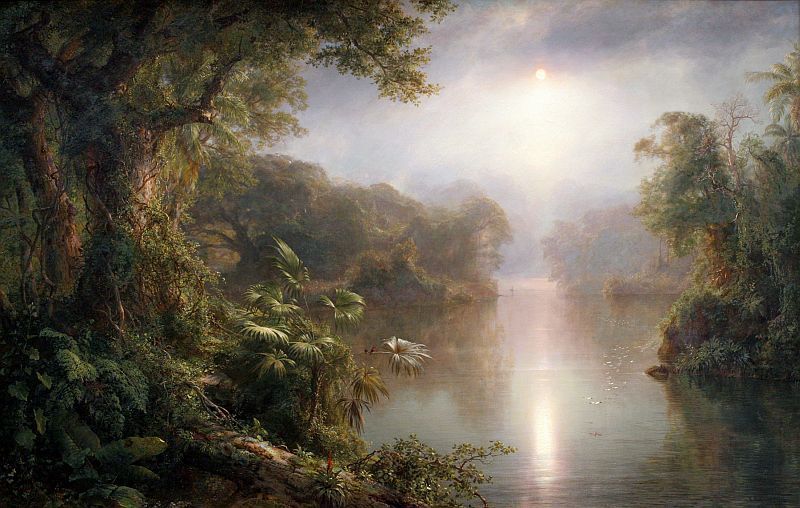This impressionistic oil painting, titled "The River of Light" (El Rio de Luz) by Frederick Edwin Church, created in 1877, is oriented in landscape fashion and depicts a tranquil, outdoor scene. The painting features a body of water, possibly a small lake, pond, or even a swamp, with water that is a somber brownish-gray rather than a vibrant blue or green. The sky above is clouded, with the sun faintly visible in the upper right portion, casting a soft white reflection on the water's surface. Majestic trees with various types of foliage, including those resembling long, palmy leaves, frame the scene, some leaning and arching gracefully over the water. Vines dangle from the branches, adding to the dense, verdant, and slightly wild atmosphere. Additional trees and vegetation recede into the distance through a gap along the body of water. The painting is characterized by a palette of dark greens, browns, and grays, enhancing the impressionistic style that captures the reflective quality of the light and the serene yet moody ambiance of the natural setting.